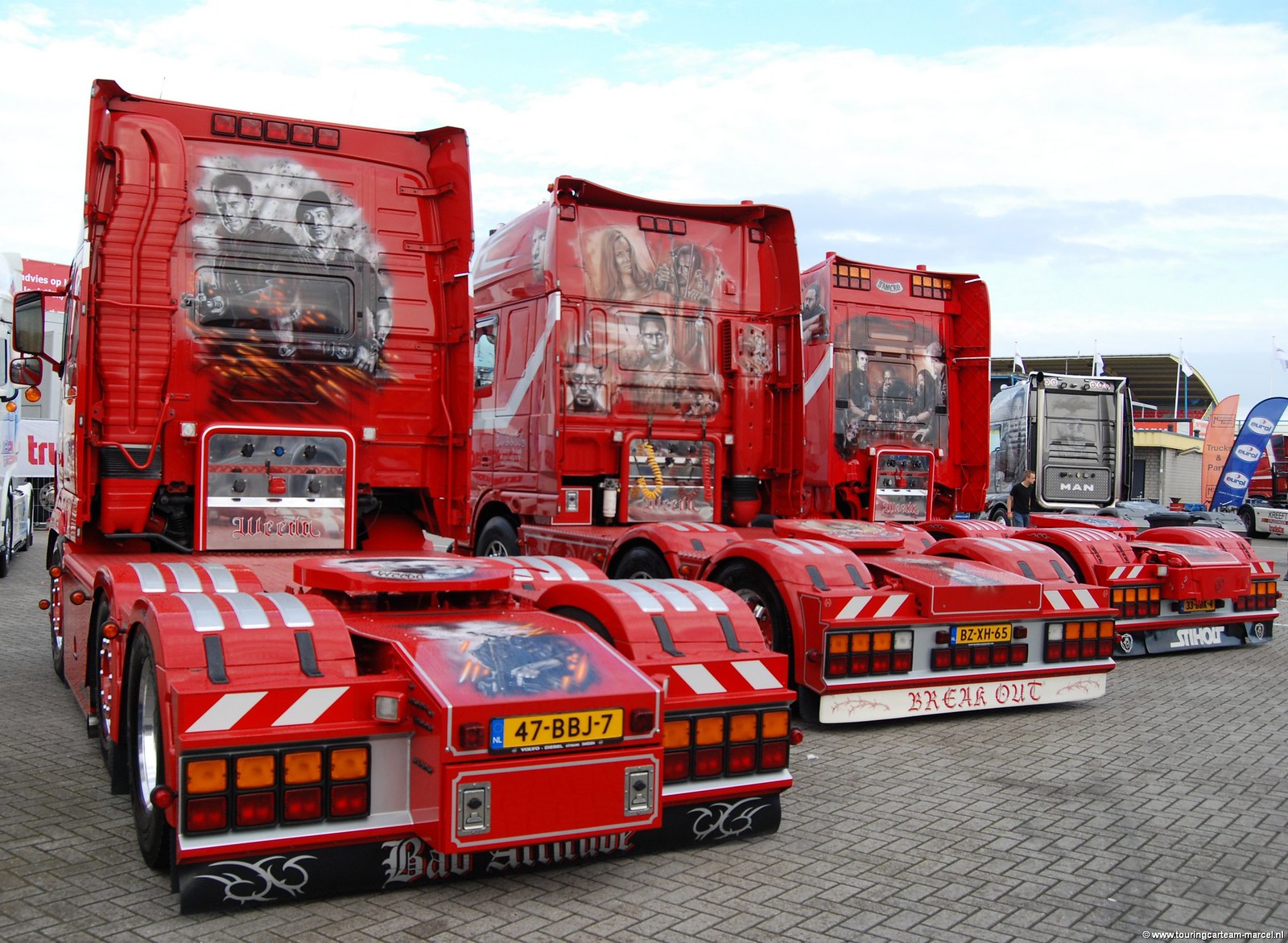This is a landscape colour photograph taken outdoors, showcasing the rear view of three vibrantly painted semi-trucks, predominantly red. Each truck features eye-catching black and white images painted on the upper rear sections, depicting scenes that resemble movie posters—one identifiable as a scene from "The Expendables" and another showcasing stylized drawings of various notable figures. The middle truck prominently displays the slogan "Break Out" in red on a white background near its base. The trucks are lined up side by side on a grey paved area composed of crisscrossed bricks, and each conspicuously bears a yellow number plate with blue edges; the nearest plate reads 4788JT. The backdrop shows a partly cloudy sky with patches of blue and a large structure with indistinct writing, possibly indicating a fairground setting. A man can be seen walking between the trucks, hinting that this might be a truck show.